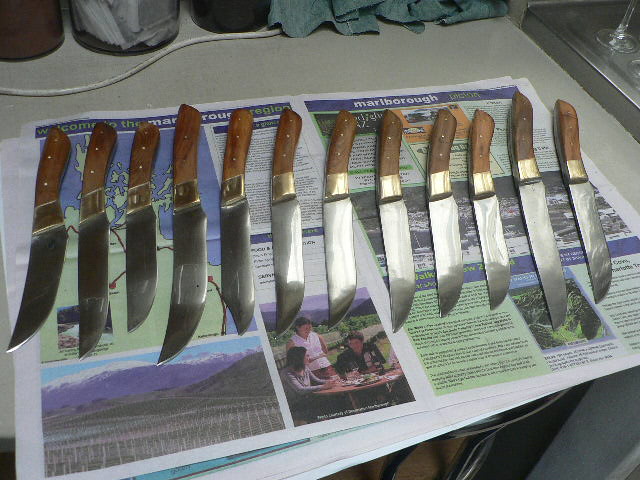The image features an indoor setting, possibly in a kitchen, with a detailed arrangement of objects. Central to the image is a flat, gray surface covered by a spread-out newspaper. The newspaper, which prominently displays the word "MARIBOROUGH" on both sides, features a map on its left side. Laid out meticulously in the middle of the newspaper are 12 knives, each with medium brown wooden handles and silver blades. The handles are encircled by a gold band at their base. While the knives' handles are uniform, their blades vary in shape, suggesting they are part of a hunting or utility set rather than kitchen knives.

To the top right of the image, a glimpse of a metal structure is seen, atop which rest two glass cups, each supported by a long pillar. Moving left from this structure, there are three bottles, one of which is conspicuously filled with white paper. Further left, a light dark blue cloth, possibly a shirt or dish towel, is partially visible. The overall scene, captured as if taken by a phone, emphasizes the alignment and variety of the knives while subtly highlighting other household elements in the background.